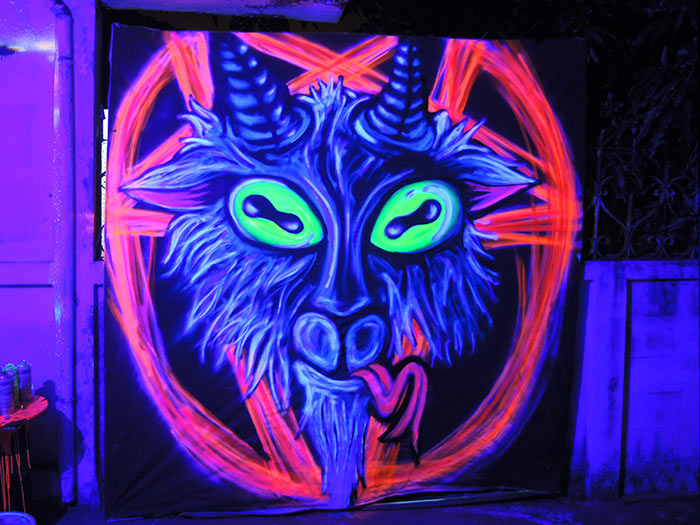The image depicts an elaborate piece of graffiti art featuring a vividly illuminated goat's head with an otherworldly neon glow. Central to the image is the goat's bluish-colored face with shaggy fur and sharply pointed black horns adorned with ring-like lines. Its eerie glowing green eyes, teardrop-shaped with black infinity-sign-like pupils, peer out menacingly. The goat's nose has large flaring nostrils, and its tongue is vividly pink, curling and split at the end, hanging out over a long billy goat goatee. Surrounding the goat’s head is a red pentagram, drawn with multiple overlapping lines that forms a rough circle. This pentagram has a vibrant but sketchy neon quality to it, accentuating the supernatural theme.

The background is dark, possibly indicating a dimly lit alley or an indoor setting under blacklight, enhancing the purplish-neon reflection from the painting. Nearby, a round table cluttered with spray paint cans sits at the left, evidence of the artwork's creation. The setting includes elements suggesting an urban environment, such as distressed furniture and possible features like a gate or garage, contributing to the gritty, nocturnal atmosphere. This ghostly and vibrant image manages to blend street art with a surreal, almost Satanic edge, symbolized by the Baphomet-like goat enveloped in its glowing pentagram.